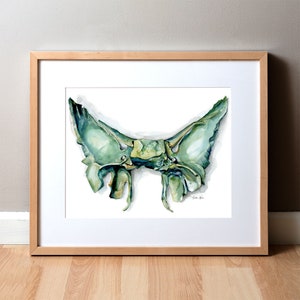The image captures a framed painting propped against a gray wall with white trim, resting on a light-colored wooden floor. The painting is encased in a light wood frame with a thick white matting board, accentuating the artwork, which is set on even whiter paper. The green-hued subject of the painting, reminiscent of a frog, features a frog-like head with two eyes and a mouth in the center. It has appendages that could be interpreted as wings, showing varied shades of green from light, almost white, to a yellowish green. The overall shape hints at a butterfly, with curved wing-like extensions and two leg-like appendages at the bottom. The image presents an intriguing blend of frog and butterfly characteristics, creating a captivating, amphibian-like figure.